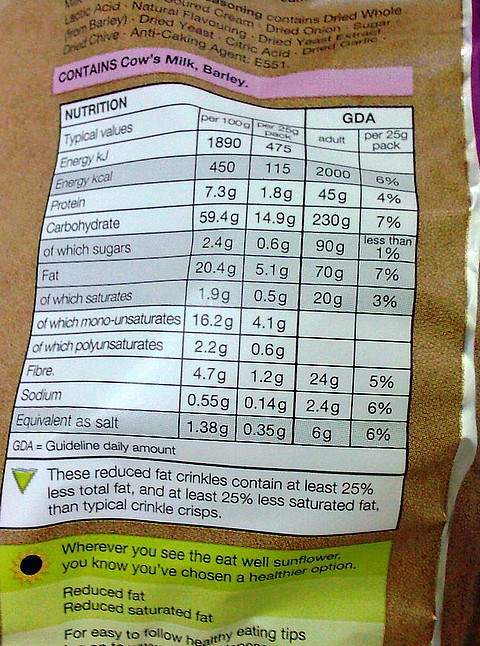The back of the food packaging features a dark brown background with a detailed listing of nutritional values and ingredients. At the top, the visible ingredients include dried onion, sugar, dried yeast, citric acid, dried garlic, dried chive, and an anti-caking agent labeled as E551, although the list is partially cut off.

A prominent purple bar highlights allergen information, stating "Contains cow milk and barley." Below this, the nutritional information is organized into two columns: "Nutrition" and "GDA" (Guideline Daily Amount). The "Nutrition" column provides typical values for energy (both in kilojoules and kilocalories), protein, carbohydrates (with a sub-category for sugars), fats (with sub-categories for saturates, monounsaturates, and polyunsaturates), fiber, sodium, and salt equivalents.

The packaging also promotes the product as a healthier option, noting that these reduced-fat crinkles contain at least 25% less fat and 25% less saturated fat than typical crisps. An emblem featuring the "eat well sunflower" signifies a healthier choice.

Rows of nutritional data detail the values per 100 grams and per 25-gram pack, including percentages of the recommended daily amounts for adults. Additional messaging offers easy-to-follow healthy tips aimed at reducing fat and saturated fat intake.